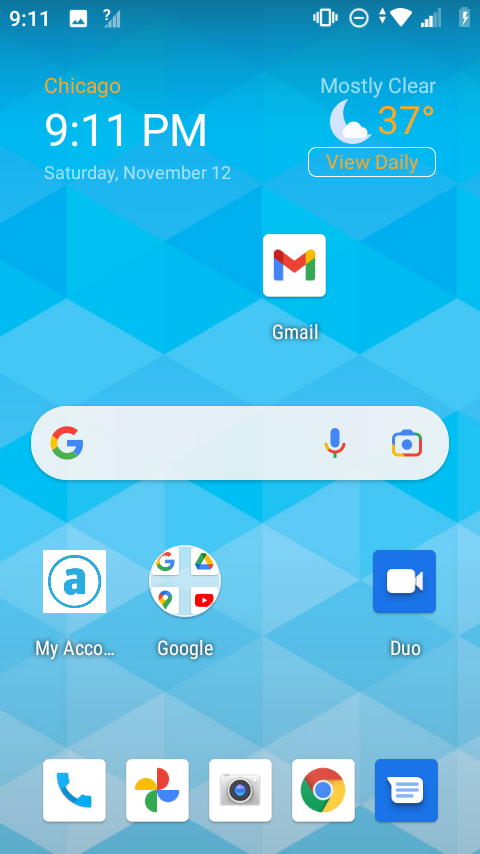**Detailed Caption:**

The screenshot captures the home page of a smartphone, displaying an intricate blue diamond-patterned background. The diamond shapes stretch horizontally and alternate between dark blue, light blue, and a mixed hue, creating a visually appealing gradient effect. 

In the top right corner, white text indicates the time as 9:11 PM. Beside it, an icon suggests that a picture is being displayed. Adjacent to this is the four-bar signal strength icon with a question mark overhead, and next is an icon indicating the phone is on vibrate mode, depicted as an outlined phone with vibration lines. Following these icons is a circle with a line through it, representing the "Do Not Disturb" mode. To its right are small arrows pointing upward and downward, denoting data synchronization. The Wi-Fi icon is illuminated white, showing three out of five bars, and the battery icon next to it indicates that the battery is currently charging. 

Below the status icons, the home screen features the current date and time in yellow: "Chicago, 9:11 PM, Saturday, November 12th." To the right, it mentions a clear weather status with a half-moon and a small cloud icon. The temperature is displayed in yellow, reading 37°F, with an option to "View Daily" below it.

Further down, the home screen contains several apps and widgets:
1. A Google Mail (Gmail) icon.
2. A Google search bar.
3. A square icon with a blue circle and a small white 'A' inside, labeled "My Account."
4. A circular Google app icon with a grouping of various Google services, labeled "Google."
5. A blue box with a white camera icon labeled "Duo."

At the bottom of the screen is a dock containing five essential app icons:
1. Phone
2. Photos
3. Camera
4. Google
5. Messaging

This detailed layout provides a clear representation of the smartphone's home page, showcasing the user's organizational structure and aesthetic preferences.